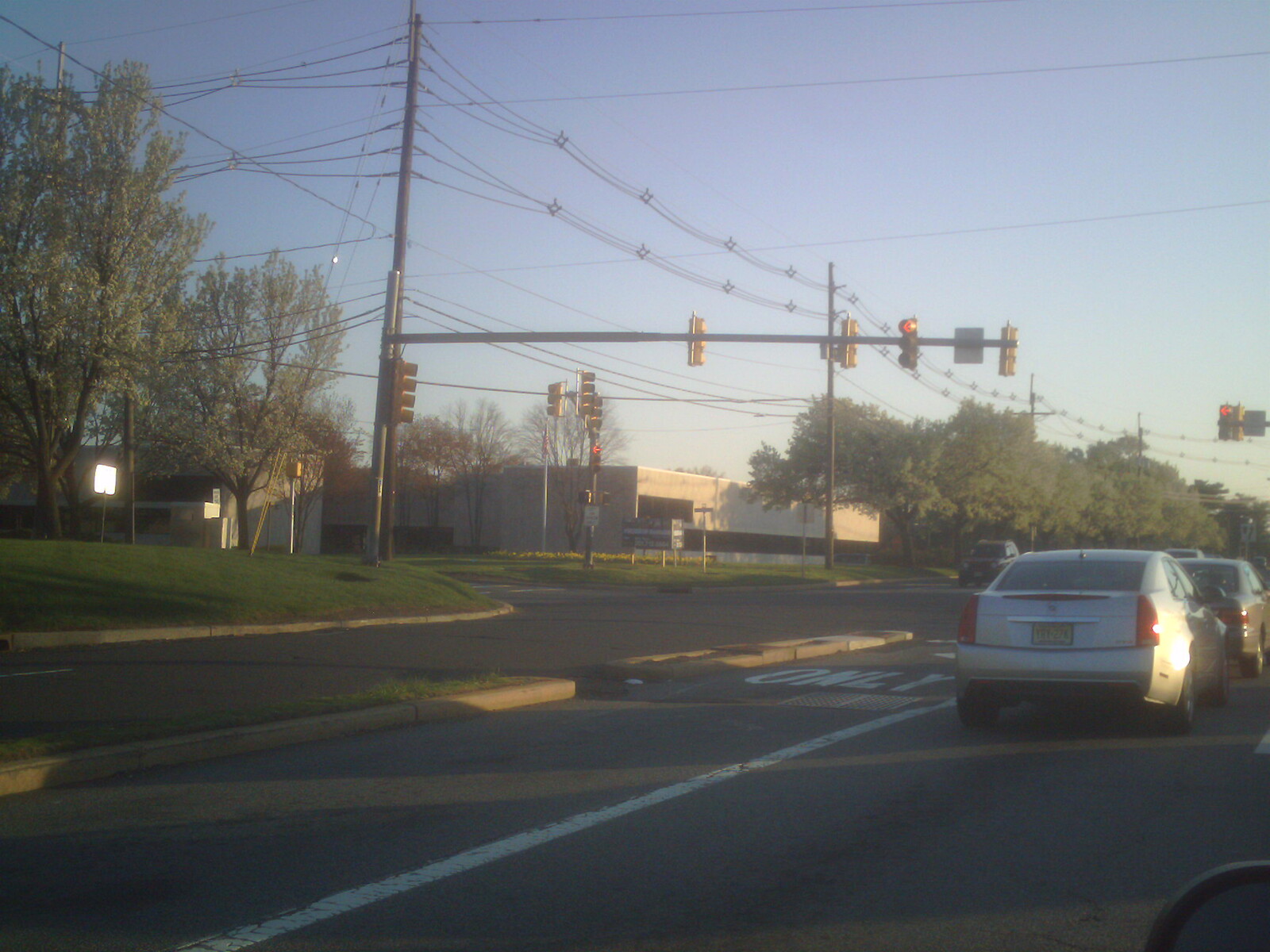The photograph captures a traffic intersection at sunset, taken from inside a car, possibly through an open window. The sky is a calm blue, indicative of the setting sun. In the foreground, two cars are visible in the adjacent lane: a dark grey sedan in front and a silver Cadillac behind it. Both are stopped at a red traffic light. There are white lane markings on the road, including the word "ONLY" written in white on the left side of the street. The intersection is a four-way crossing with multiple lanes, including a possible bus lane on the right-hand side. On the far left lane, a white van is partially visible. The sidewalks are bordered with grass, and various buildings and additional traffic lights are visible in the background. The traffic lights are suspended from a metal pole extending across the intersection, ensuring they are visible to drivers approaching from a distance.